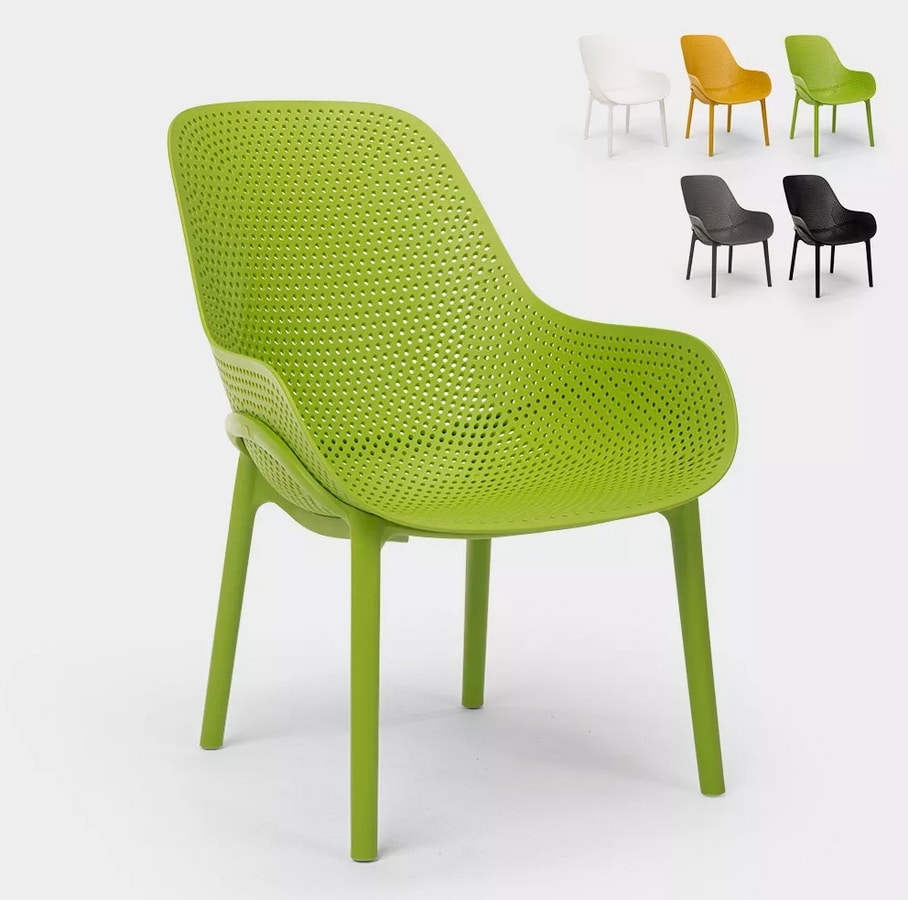The image features a prominently displayed lime green chair with a unique design, characterized by its all-plastic construction and numerous holes that give it a mesh-like appearance, indicating breathability suitable for outdoor use. The chair, placed centrally in the foreground with four solid, straight cylindrical legs, stands out against a solid white background. In the top right corner, there are smaller representations of the same chair model in different color variations including white, light orange, lime green, charcoal gray, and black. The image provides a clear, detailed view of the chair's design and available color options, presented in a square format without any accompanying text.